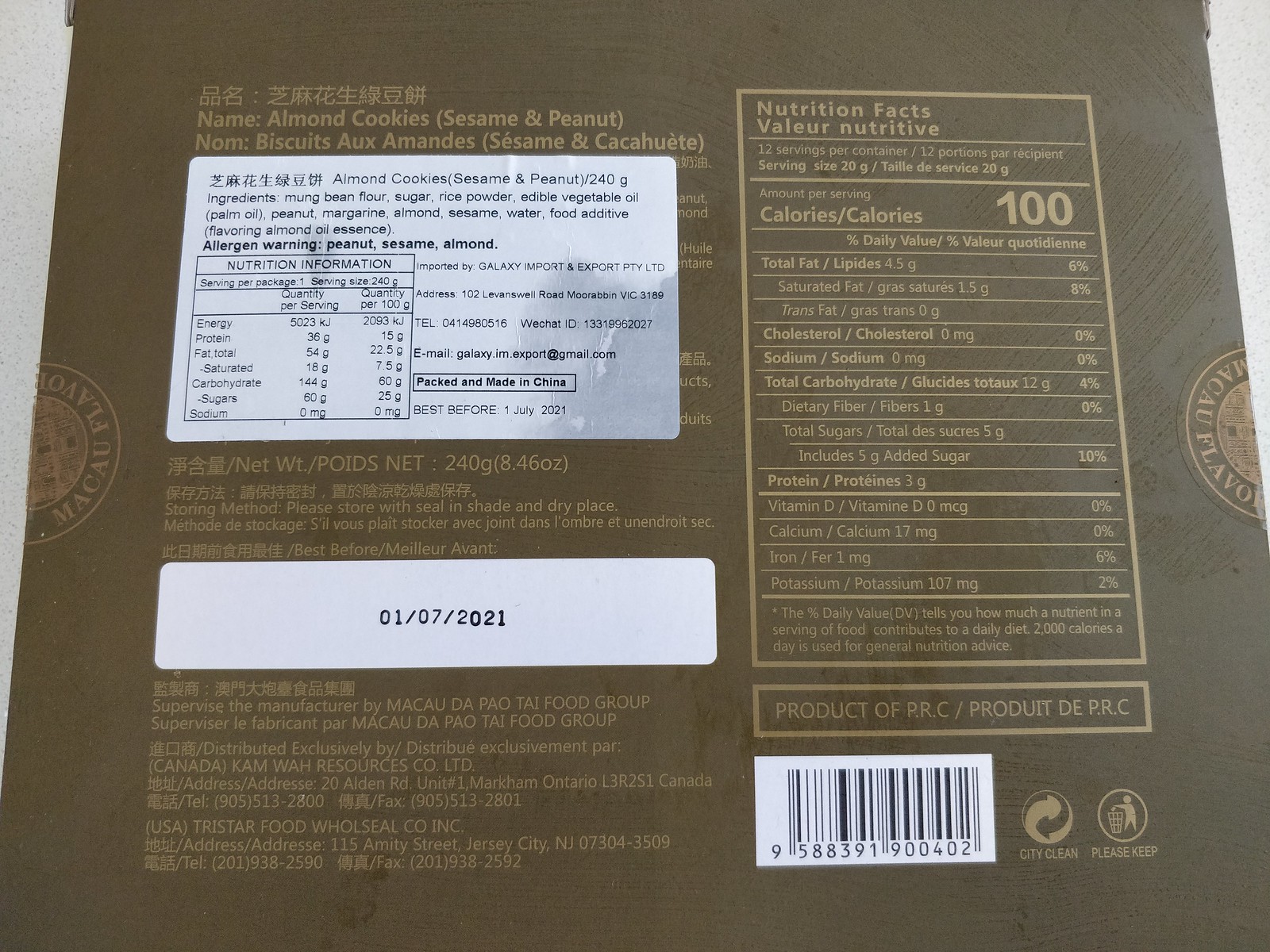This photograph captures the back of a package of cookies, specifically showcasing its detailed labeling and design. The packaging, predominantly dark brown, is adorned with elegant gold text. On the left side, the product name “Almond Cookies” is displayed prominently, with additional flavor details in parentheses—“sesame and peanut.” The left section also features a white rectangular area containing the nutritional information and ingredient list, clearly printed in black text.

Central to the left side is the expiration date, marked as 01/07/2021. The right side of the package exhibits a large gold rectangle, housing detailed nutritional facts including the amounts of total fat, cholesterol, sodium, and total carbohydrates. Below this, in a longer gold rectangle, the words "Product of PRC" are displayed.

Towards the bottom of the package, a white background highlights a black barcode, flanked by several logos indicating the product’s cleanliness and recycling information. This meticulous presentation of information ensures the consumer is well-informed about the product's contents and origins.